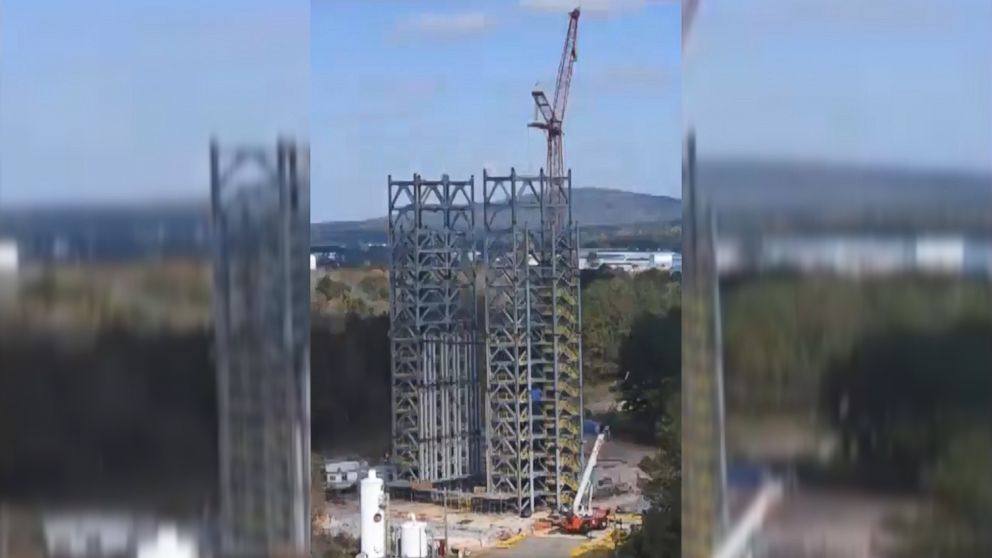The photograph prominently captures an active construction site in the midst of a picturesque outdoor setting. The image is rectangular, measuring approximately six inches wide and three inches high, with only the center third clear and the left and right thirds blurred, giving the composition a unique aesthetic. At the core of the image, a multi-story building is in the early stages of construction, featuring extensive grey steel scaffolding and metal framework. Behind the framework, a large red crane towers over the construction site, assisting in the assembly of the structure. A smaller crane and a small hut are observable at the lower part of the image. In the background, a serene landscape of trees, cityscape elements, and a mountain range unfolds under a blue sky dotted with grey clouds. The blurred sections to the left and right still reveal parts of the construction and the surroundings, including indications of additional steel structures and a red vehicle equipped with a white area lift. This striking image juxtaposes the ruggedness of construction with the tranquility of nature.